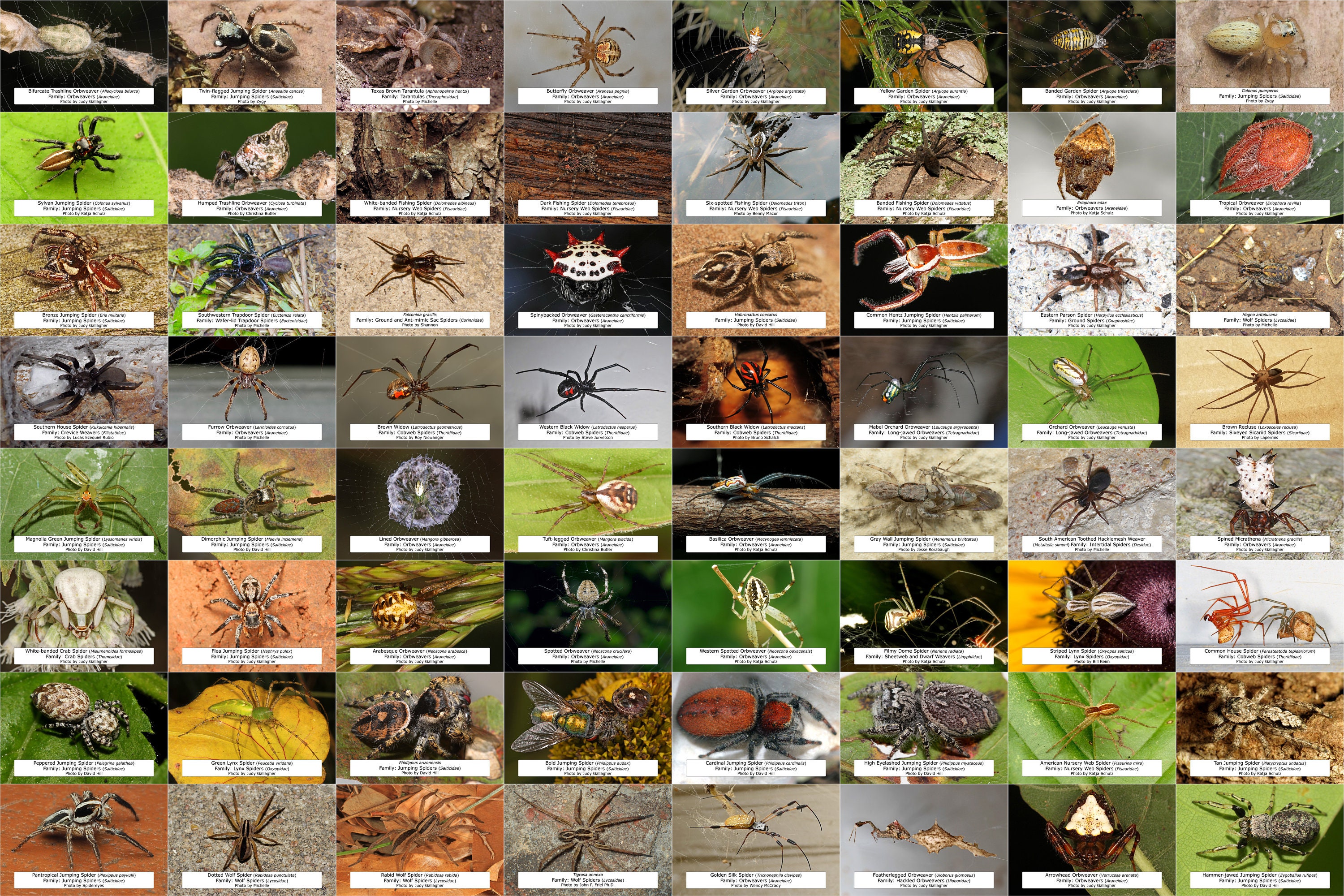This image displays a poster classifying spiders, featuring approximately 50 to 64 postage stamp-sized photographs of various arachnids. Each tiny image contains a distinct spider, positioned against diverse backgrounds such as spiderwebs, green and yellow leaves, boards, or the ground. The spiders exhibit a range of colors including black, white, red, black and red, and beige. Under each spider, there's a small white box with barely legible black text that likely provides the common and scientific names of the spiders. The meticulously compiled images present a detailed taxonomy of spider species, showcasing their variation in shape, size, and hue.